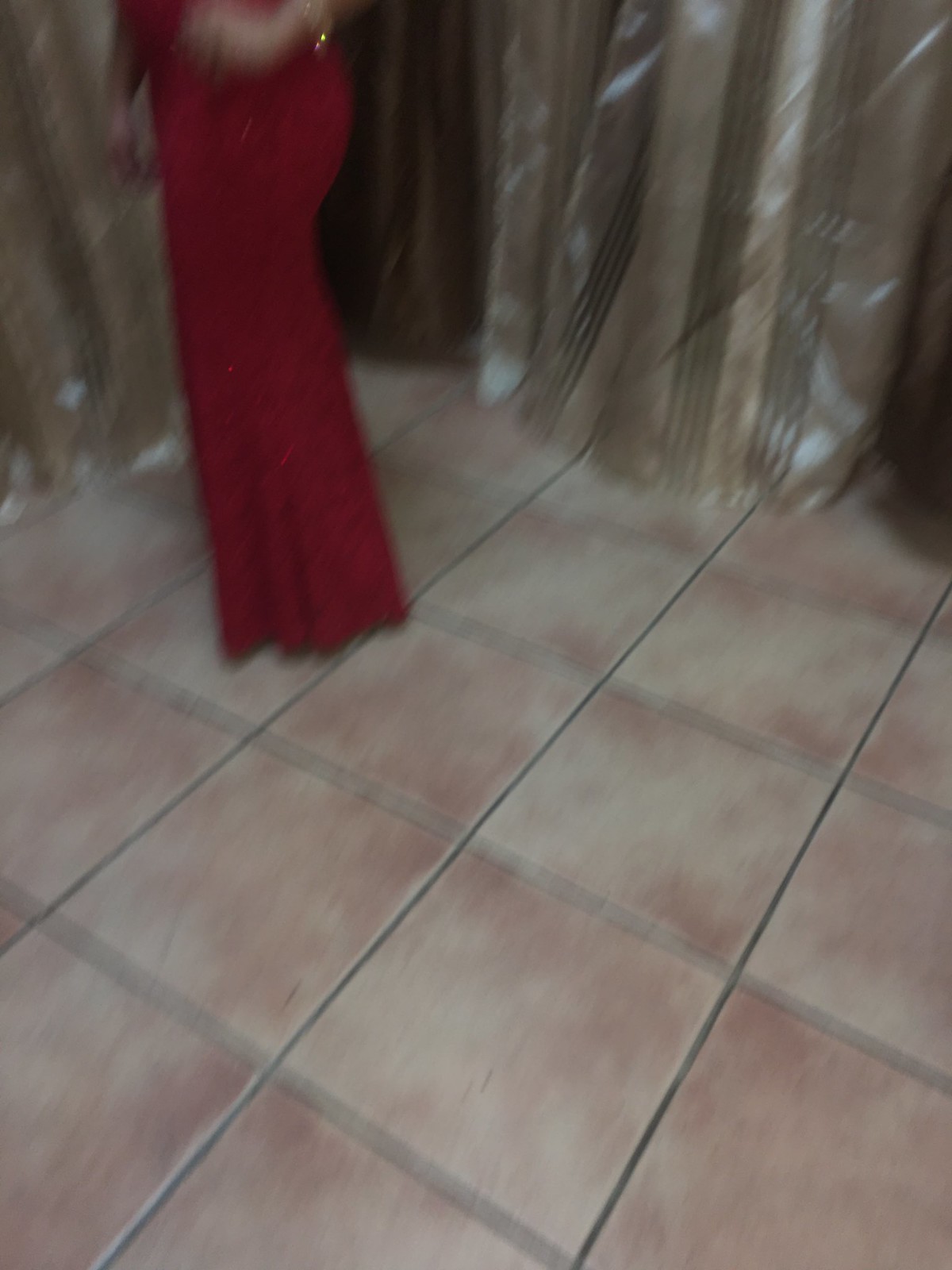The image depicts a top-down view of a tile floor composed of square tiles in shades of reddish-brown and white. In the upper left corner of the image stands a Caucasian woman who appears to be donning a wine-red, sparkly ball gown that fits snugly around her thighs and buttocks before flaring out with pleats at the bottom. The dress reaches down to her feet, obscuring her shoes. Her arms hang down by her sides, and she has either brown hair or is holding something with brown fur, possibly a boa. In the background, which lacks walls, there are vertical-striped, almost see-through plastic curtains adorned with brown and gold stripes. These curtains create a rectangle-like shape, enhancing the impression of an enclosed space or stage. Additionally, there is a blurry patch of white fur near the woman's left side and a subtle hint of a gold accessory on her left arm. The overall scene exudes a sense of elegance and mystery, framed within a distinctly tiled setting.